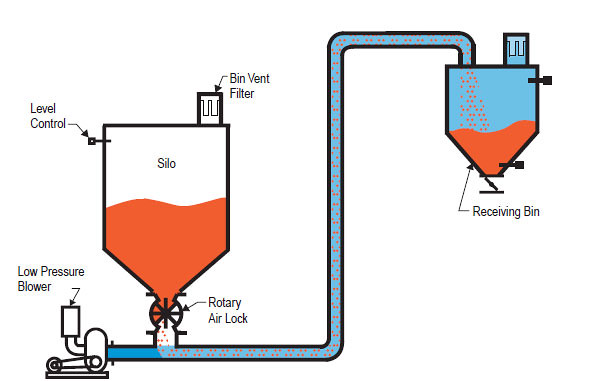This detailed schematic depicts a cartoonish representation of a silo system, illustrating the flow and processing of materials. The prominently white and orange silo on the left, shaped somewhat like a trapezoid with a flared bottom, features a "bin vent filter" labeled at its top and a "level control" on its left side. Enlarged words identify these components, adding to the clarity of the drawing. 

At the base of the silo, there is a "rotary air lock," a valve-like mechanism that regulates the release of the stored material. Connected to this air lock is a blue pipe—bright and vibrant—highlighting the flow path of the material through the system. Along the horizontal part of this tubing, near the base of the silo, is annotated "low pressure blower," indicating a device that aids in the material's movement through the pipe.

The pipe extends from the rotary air lock, taking a convoluted route: first heading to the left, then rising above the silo, moving horizontally to the right, and finally descending into a "receiving bin," which mirrors the design of the silo but is comparatively smaller. This receiving bin is similarly labeled with a "bin vent filter" at its top.

Inside the pipe and receiving bin, orange dots travel and accumulate, signifying the material flow from the silo to the receiving bin. The lower half of both the silo and the receiving bin is filled with the orange substance, contrasting with their white upper halves, to visually represent the half-filled state of the containers. The blue pipe's bright hue makes the movement of orange grains especially noticeable, depicting a clear, continuous path of the material as it is transferred from the silo to the receiving bin.